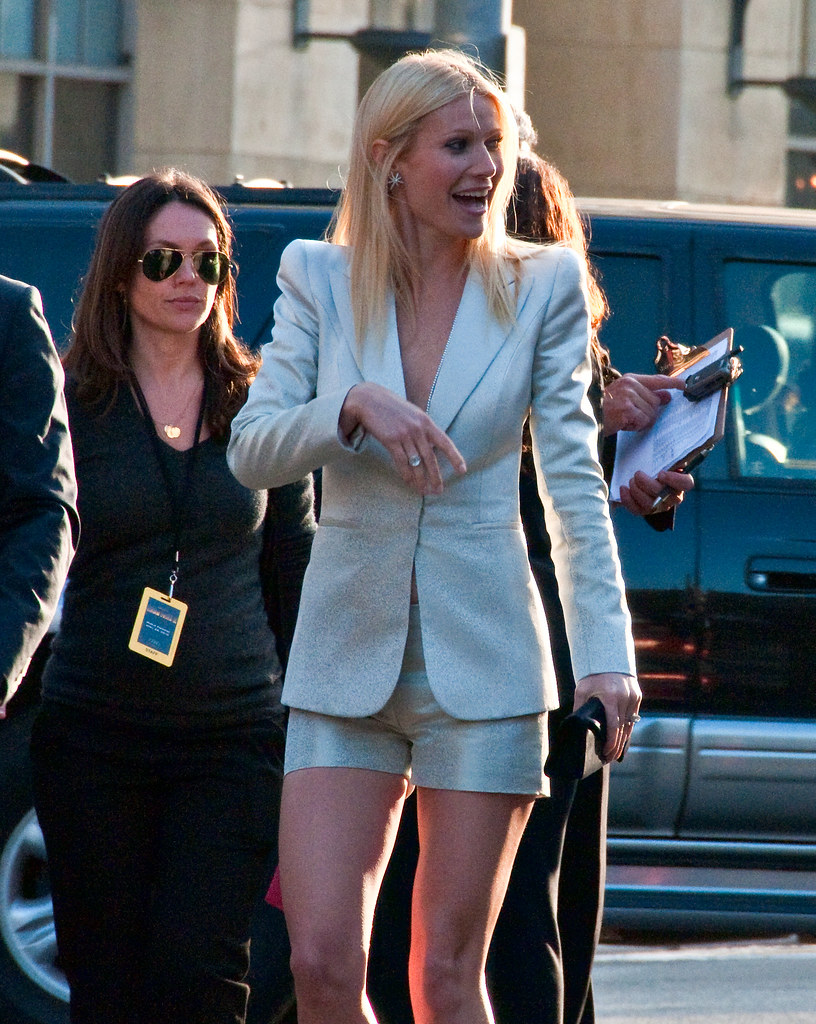In this daytime image, actress Gwyneth Paltrow is strolling outdoors, possibly to an event or down a street. Gwyneth has straight, chest-length blonde hair and is adorned with light-colored Starburst earrings. Her outfit consists of an off-white, silvery suit jacket with no shirt underneath, paired with matching shorts, giving her a tall, slender appearance. She carries a small black clutch purse in her right hand and is looking to her left with her mouth slightly open.

Several people are around her, seemingly aides or bodyguards. One woman behind her, with straight brown hair and sunglasses, wears a black shirt and pants, accessorized with a lanyard that has a blue and gold tag. She has a serious, perhaps annoyed expression. Another woman nearby holds a clipboard with white papers. The scene includes a black SUV and a tan building with windows in the background, with the sunlight casting a bright glow on the edge of Gwyneth. The overall atmosphere suggests a high-profile event or arrival.